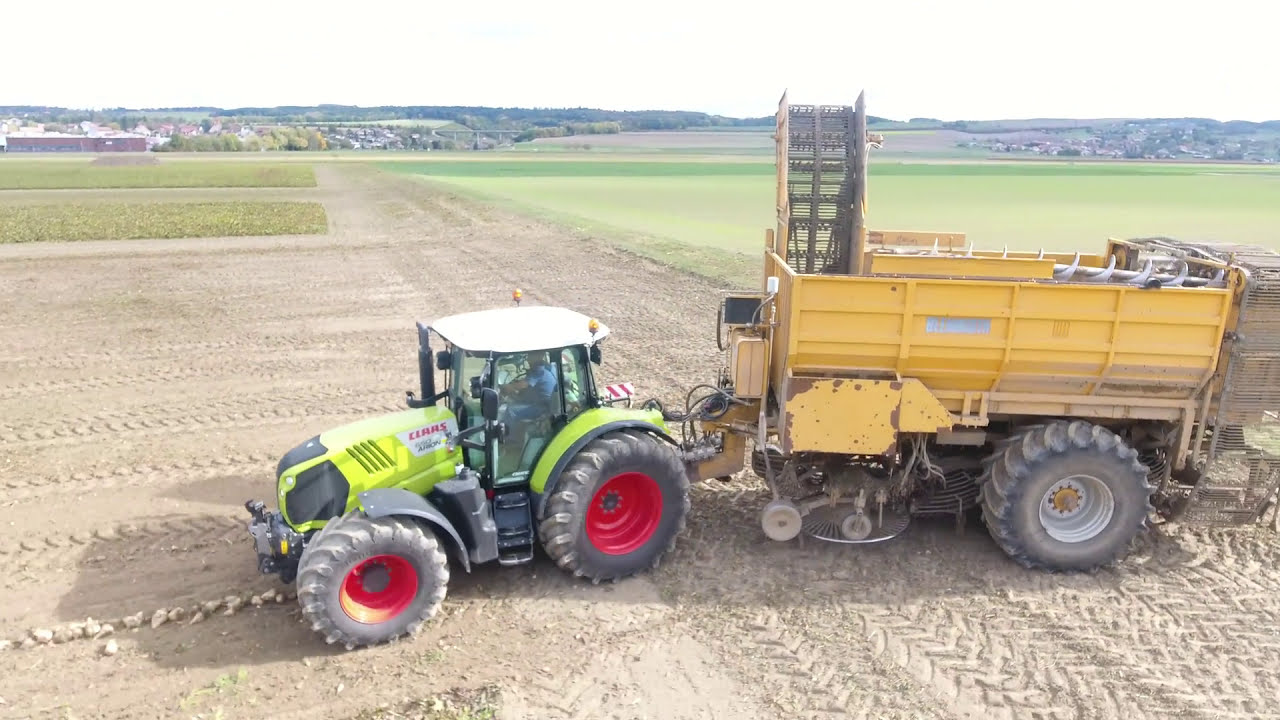The image depicts a vibrant farm scene with a neon yellow tractor, featuring red wheels and a green body with "CLAAS" written in red text on the back of the engine casing. The tractor has a white roof with two orange lights and a glass-enclosed cabin where a man wearing blue is driving. It tows a large yellow piece of farm equipment with a grid pattern, large rear rubber pneumatic tires, and a spiral drill loaded into the back. The foreground showcases dry soil marked with tire imprints, while the background transitions into green pastureland on the right and an agricultural structure on the left. The horizon is dotted with small buildings, houses, trees, and distant hills under a light sky.